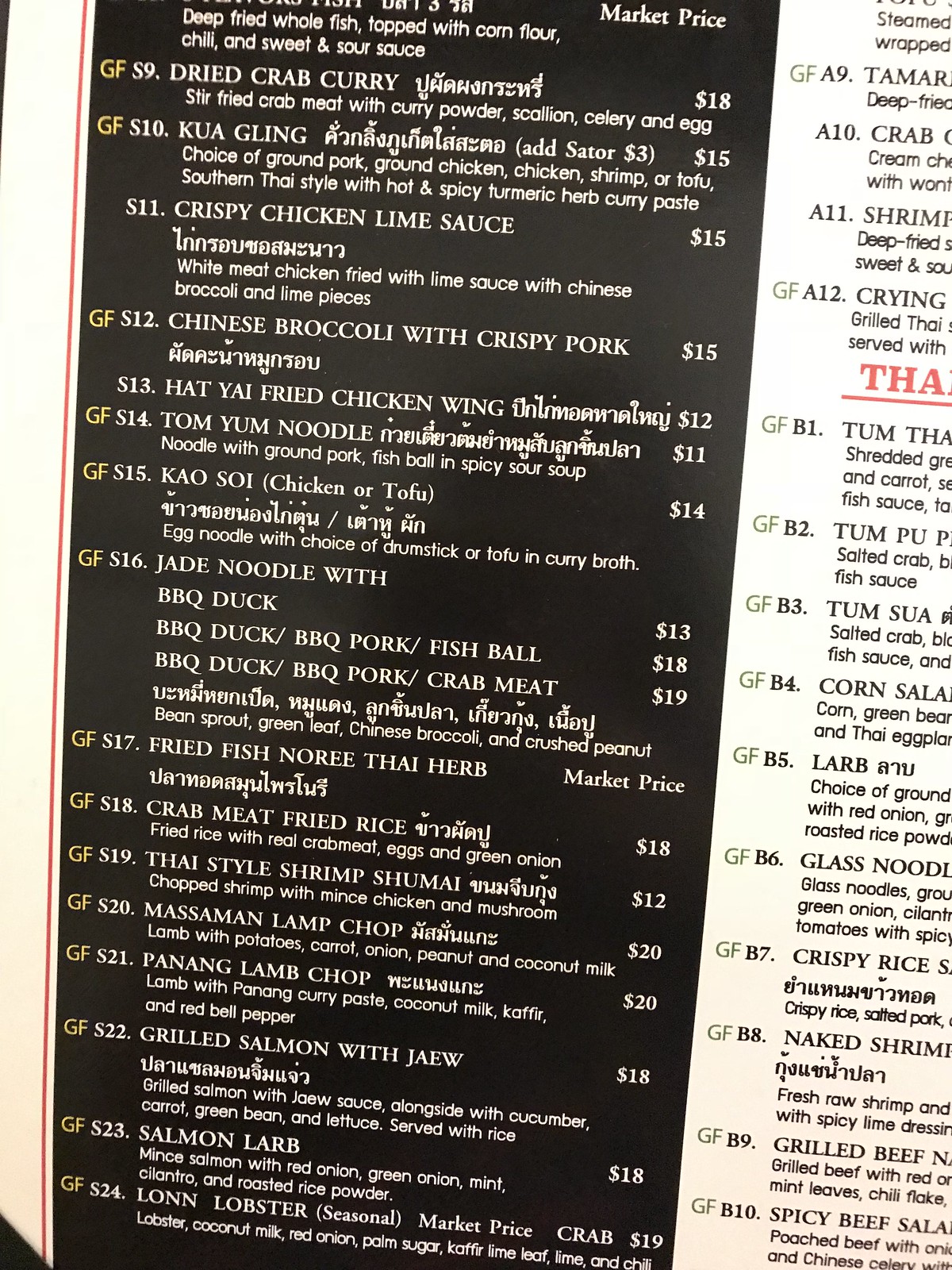The image reveals a restaurant menu brimming with an extensive array of culinary delights. Prominent items on this menu include a delectable Dried Crab Curry priced at $18, a flavorful Kua Gling for $15, and Crispy Chicken Lime Sauce for $15. Other enticing offerings feature Chinese Broccoli with Crispy Pork at $15, savory Fried Chicken Wings, and a Tom Yum Noodle Dish. The menu also boasts the exotic Khao Soi, and the intriguing Jade Noodles with Barbecued Duck, with options to add Fish Ball and Crab Meat.

Seafood lovers will delight in the bounty of choices including Fried Fish, Nori, Thai Herb Fried Rice with Thai-style Shrimp, Crab Meat, Shrimp Shumai, Panang Lamb Chop, Grilled Salmon with Jowl, Salmon Larb, and Lawn Lobster. The presentation of the menu is equally noteworthy; the right page of the menu features a pristine white background with black lettering, while the left page captivates with a sleek black background adorned with white lettering. Though some text is cut off, the menu tantalizes with mentions of other dishes like a Crispy Rice Dish, Glass Noodle Dish, Naked Shrimp Dish, and a Grilled Beef Dish, adding to the allure of this gastronomic experience.